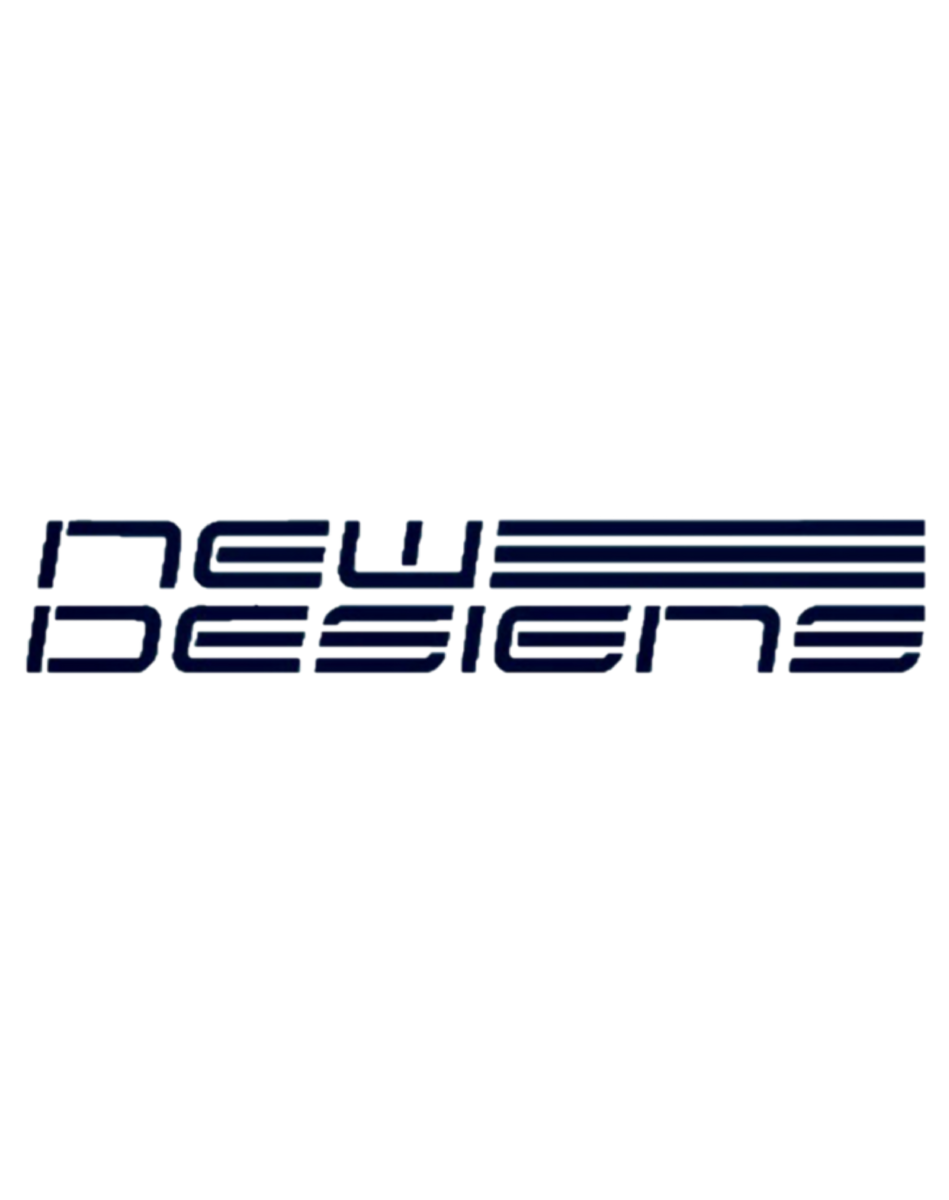The image showcases a logo for a company called "New Designs" set against a plain white background. The name "New Designs" is written in a unique and somewhat futuristic font, primarily dark blue with a silver outline that gives a reflective appearance. The design elements feature a combination of vertical and horizontal lines with rounded curves, except for the right side of the "W" in "New," which breaks this pattern. Accompanying the word "New" are three horizontal stripes of the same color and design extending from the right of the "W," aligning with the length of the word "Designs." The artistic lines create an overall cohesive and modern aesthetic, suggesting this could be a logo for a clothing company.